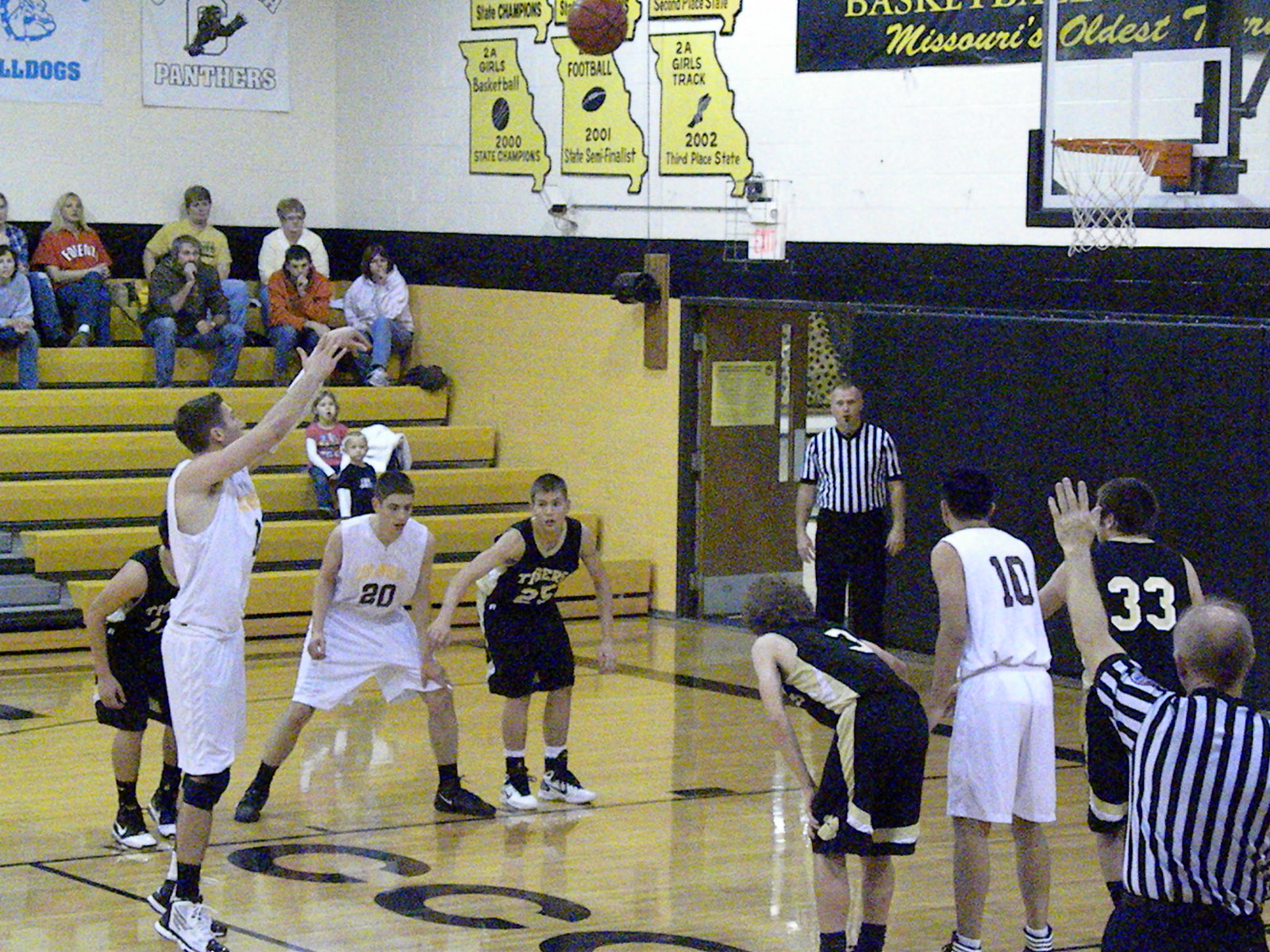This image captures a dynamic moment in an indoor basketball game played on a polished hardwood court. The scene is centered on a player, mid-jump, shooting the ball towards the hoop, which is visible in the top right corner. The teams are distinguished by their uniforms; one team wears black jerseys with black shorts, while the other dons white jerseys with white shorts. Jersey numbers such as 10, 33, 20, and 25 can be seen. 

Positioned around the central players are referees; one near double doors in the background with his back to the camera and another on the right side. Sparse but notable, the audience includes both kids and adults, men and women, seated on wooden bleachers to the left. The gymnasium is adorned with various banners; notably, ones stating "Missouri's oldest" and showcasing achievements like "2-way girls track, 2002 3rd place state," "football, 2001 state semi-finalist," and "2-way girls basketball, 2000 state champions." Logos of the teams, Bulldogs and Panthers, also embellish the background. The setting, characterized by its white and blue walls, emphasizes the energetic ambiance of an ongoing basketball game.